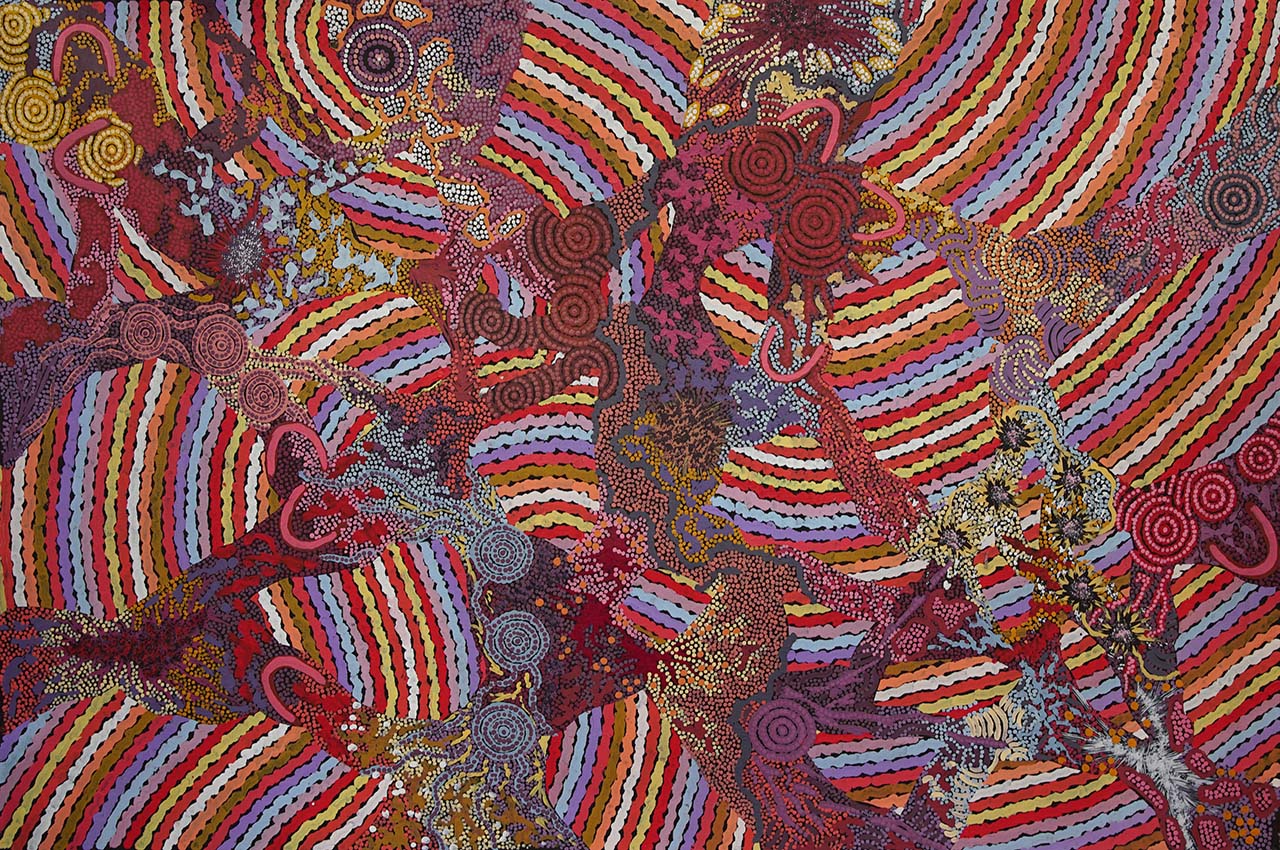This image depicts an abstract mixed media artwork, reminiscent of North African tapestry design, brimming with intricate and vibrant detailing. The overall composition features ribboning swirls of multicolored lines—blues, lavenders, purples, reds, lime greens, and whites—creating a swirling background that is both psychedelic and mesmerizing. Interwoven amid these swirling patterns are textures that form deep red, pink, maroon, and blue circles, giving the impression of embroidery-like stitches. These elements create an interconnected and layered design, with vertical and horizontal orientations of the lines and circles blending harmoniously. Amidst the tapestry-like swirl, one can discern a semblance of a female form, accentuated by two swirly red embroidery pieces that could represent breasts. The entire piece is a careful fusion of colors, shapes, and textures, resulting in a stunningly intricate and colorful work of art.